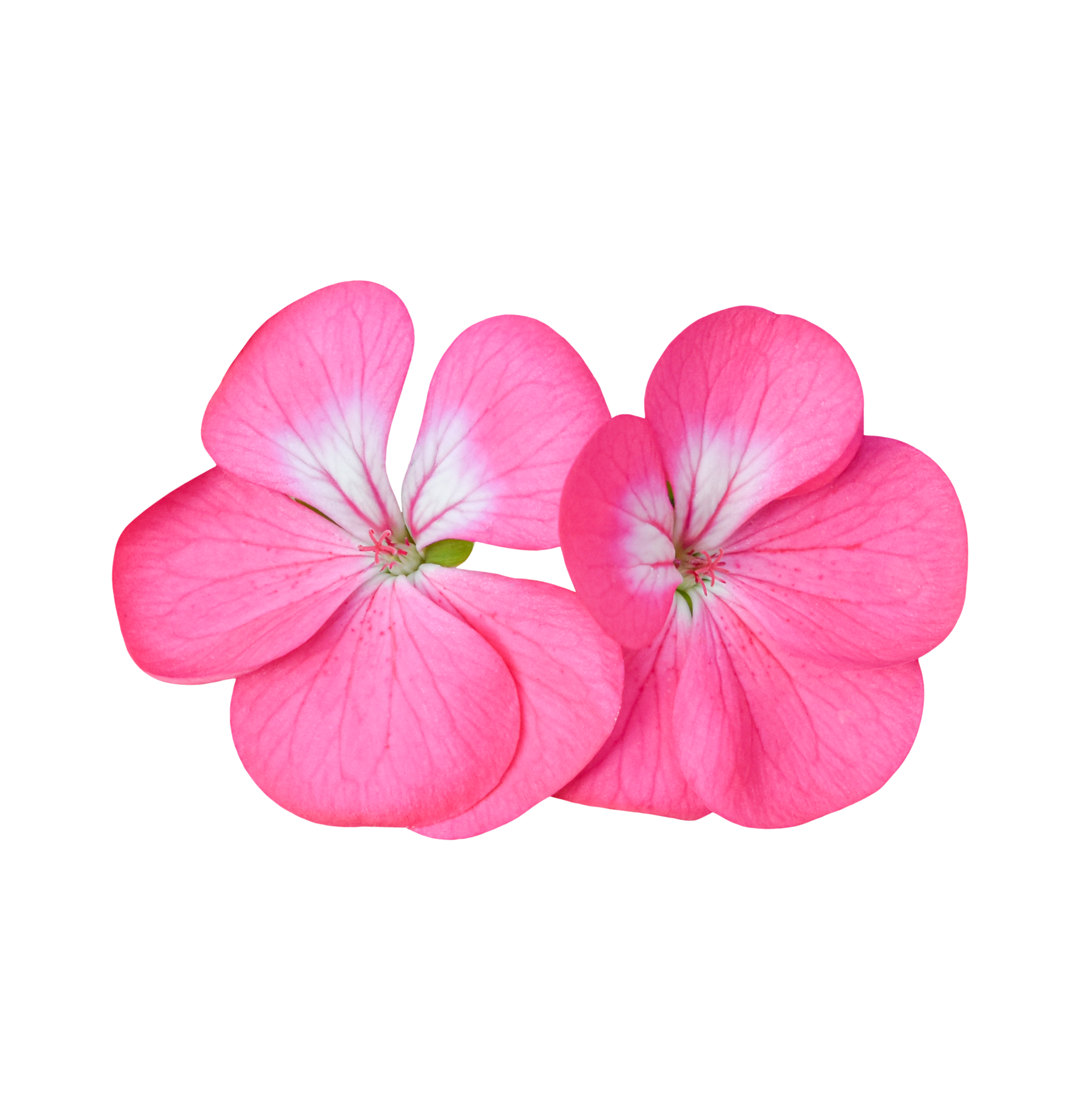This image is a detailed color photograph of two elegant and delicate pink flowers set against an all-white background. Each flower boasts multiple round petals that transition in color from a dark pink at the edges to a lighter pink, and eventually white near the center. Prominent dark pink veins run across the white portions of the petals, adding a layer of intricacy and refinement to the image. At the heart of each flower is a small green circle surrounded by protruding pink stamens. The flowers are distinct and standalone, with no visible stems, though a hint of green stem is partially obscured by the petals, and there's a leaf peeking out behind the left flower. This striking composition, featuring varying shades of pink and subtle touches of green and white, creates a vibrant contrast against the pristine white backdrop.